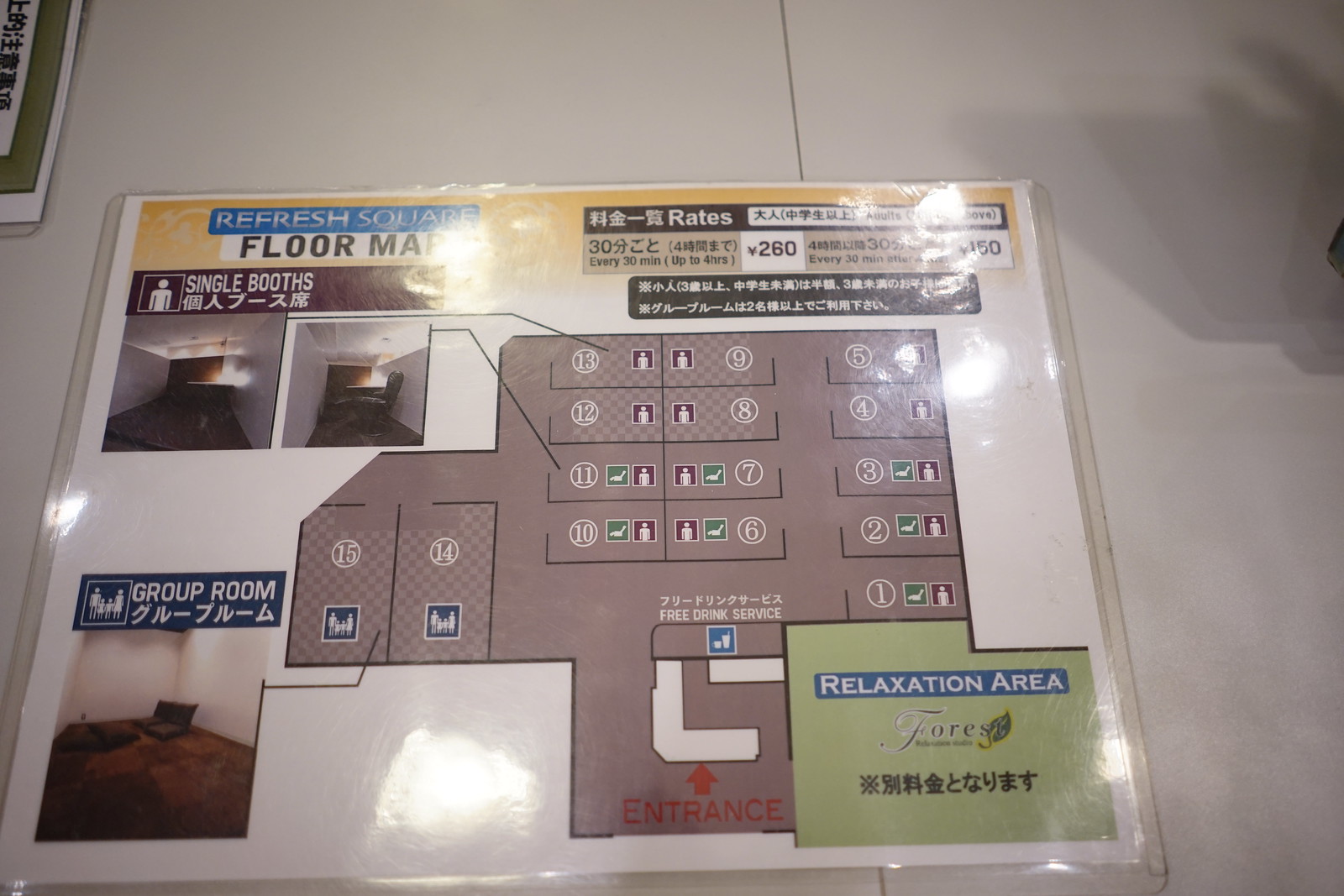This image is a detailed photograph of a laminated poster placed on a white-colored surface, displaying a floor plan of an apartment or building in an Asian country. The poster is horizontal and rectangular with a yellow bar at the very top, which has reflected light making some of the text hard to read. The top section includes a title in a blue rectangle that reads "Refresh Square Floor Map," though the reflected light partially obscures this. Adjacent to this, on the right, there is extensive text in an Asian language, detailing rates—indicated by numbers and yen symbols—implying the location is in Japan. 

The floor plan itself is prominently displayed in the middle of the poster, depicting a square design, a trapezoid shape attached to it, and a smaller rectangle below, with labels for different rooms, numbering up to 15. Photographs of the interior of the apartment or rooms are positioned on the left side and the bottom right side of the poster. The upper right section contains further unreadable text due to the light reflection, while the lower right corner specifies a "Relaxation Area Forest." The background color of the poster is predominantly white with an orange section at the top, adding a vibrant touch to the layout.